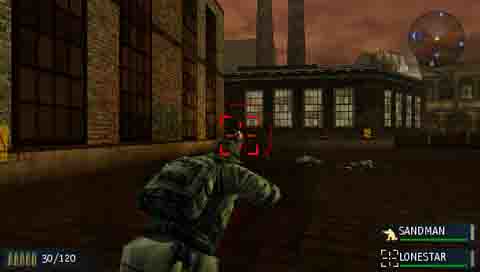This image is a blurry, dark screenshot from an older third-person military video game, potentially from the PlayStation 2 era, about 15-20 years ago. The scene is set in a factory-like environment at nighttime, with ominous reddish-brown sky illuminating the background. On the left side, there's a tall, windowless brick building, and next to it, a shorter, two-story brick building with large windows lit from the inside and two prominent smokestacks on the roof. In the foreground, we see a soldier, identified as 'Sandman,' dressed in camouflage and a backpack, aiming his gun at an enemy. The view features a red targeting reticle, indicating that 'Lone Star' is the enemy characterized in the crosshairs. At the bottom of the screen, there are indicators showing "30/120," possibly representing ammo count, along with the names 'Sandman' and 'Lone Star,' likely denoting player and enemy identifiers, respectively.